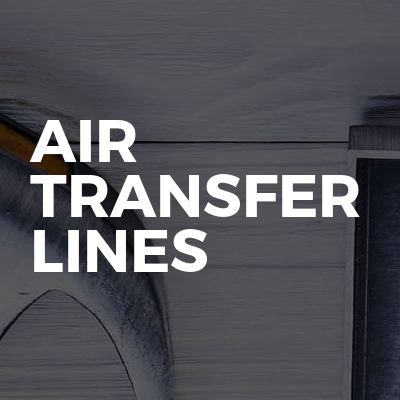In a dimly lit indoor setting, the image prominently features bold, white all-caps text saying "AIR TRANSFER LINES" arranged vertically in the center. The background consists of a wood grain texture, adding a dark, moody aesthetic to the scene. To the right, a slender, bluish post is visible, while the left side reveals a tool with a metallic texture and an orange tip resembling a hammer's claw. Nearby on the left, another object is noticeable, appearing like a white, elongated water bottle with a black rectangular label. The overall composition is abstract, with shadows obscuring finer details, giving the scene a slightly blurred and mysterious atmosphere.